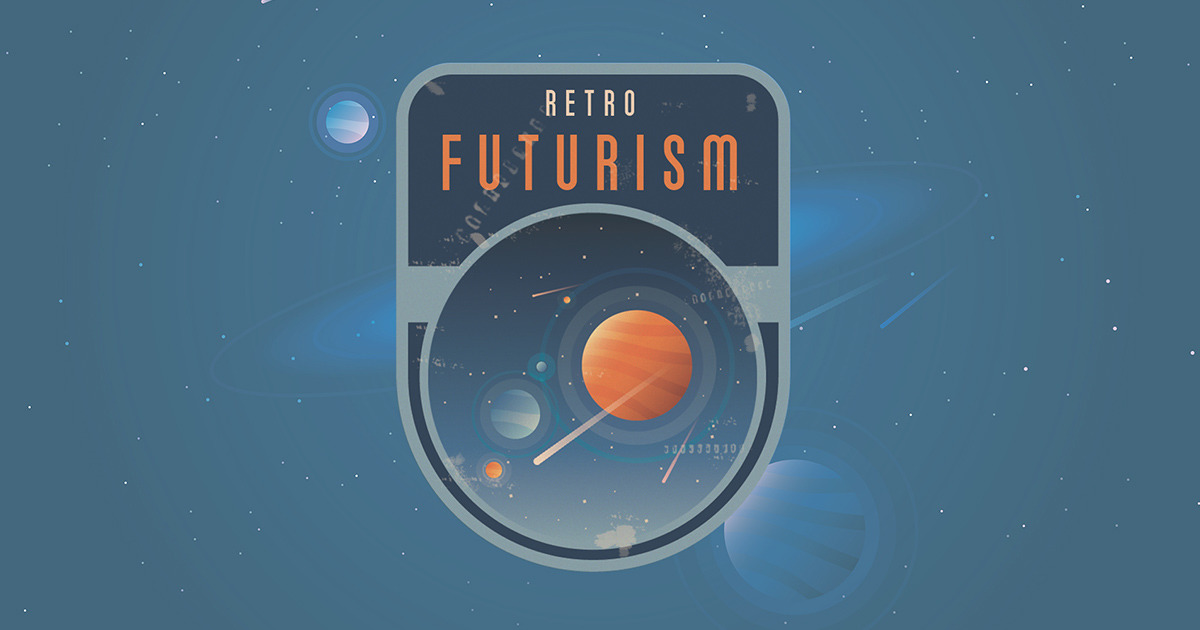The image is a digital artwork featuring a retrofuturistic theme. Central to the composition is a badge-like emblem, outlined in gray, with a flat top, curves at either side, and a semi-circular bottom. The emblem prominently displays the word "Retrofuturism," where "Retro" is written in smaller, tan or light orange letters, and "Futurism" is in a larger, bold orange font. Within the badge, there is a circle containing artistic depictions of planets, with one notably orange planet resembling Jupiter, and other celestial bodies such as stars and asteroids. The background of the image is a navy blue, resembling the night sky or outer space, dotted with specks that appear to be stars. Additional celestial elements, including what seem to be another planet at the bottom right and possible rings of Saturn, are also present. There are dynamic elements such as comets or shooting stars streaking across the scene from right to left, enhancing the space theme.